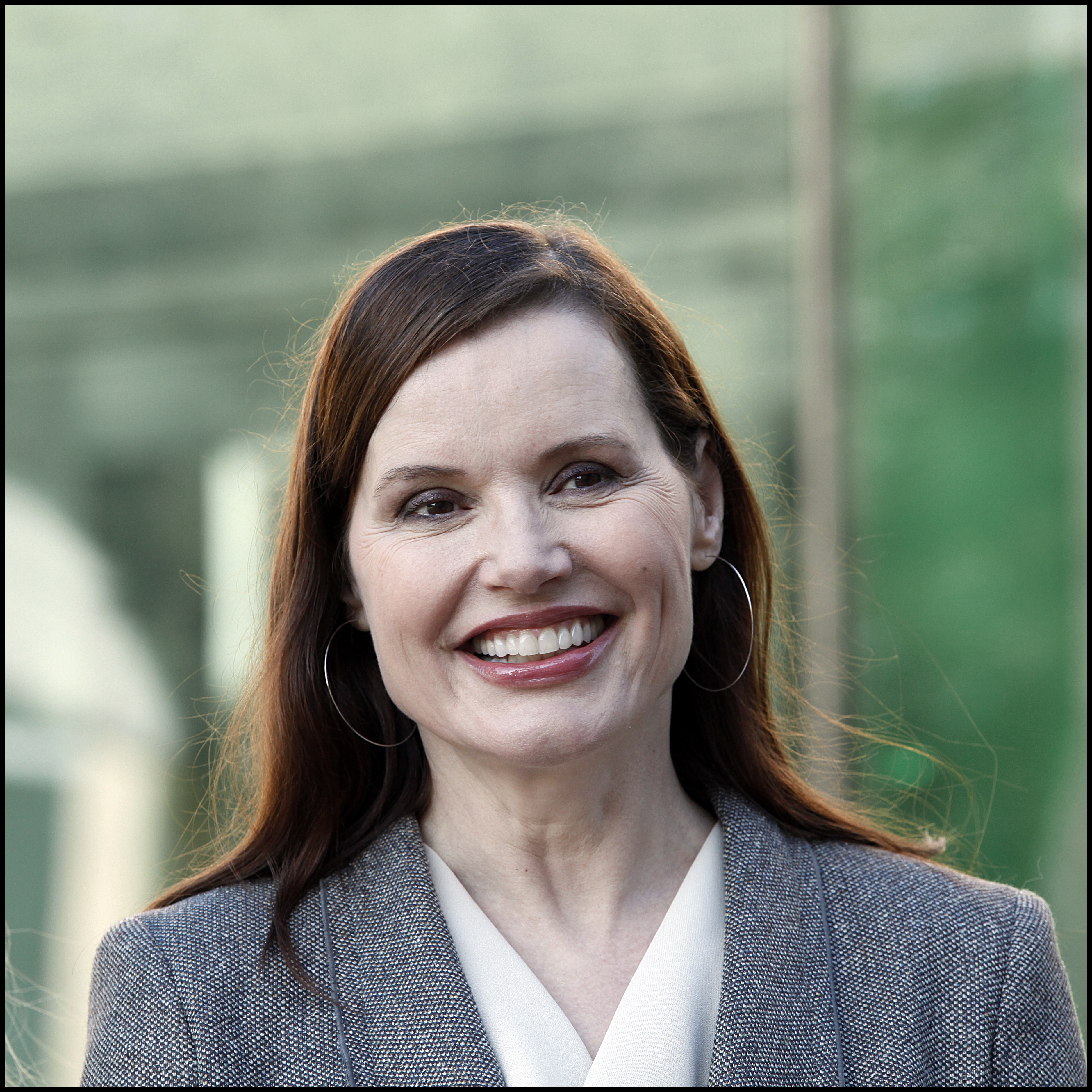The image features a close-up of a smiling older woman, likely in her 50s or 60s, with a radiant expression showing all her top teeth. She has long, straight, dark brown hair that falls past her shoulders, and her striking brown eyes are accentuated with eyeliner and gray eyeshadow. Her makeup is heavy, with noticeable red lipstick. She is dressed in a white V-neck shirt layered under a grayish-black sport coat. Large silver hoop earrings add a touch of elegance. The background is blurred, hinting at an outdoor scene with a vague structure that might be a building, bridge, or overpass, and a lot of greenery on the right side. A long vertical brown pole is also visible in the blur, enhancing the outdoor context of the setting.